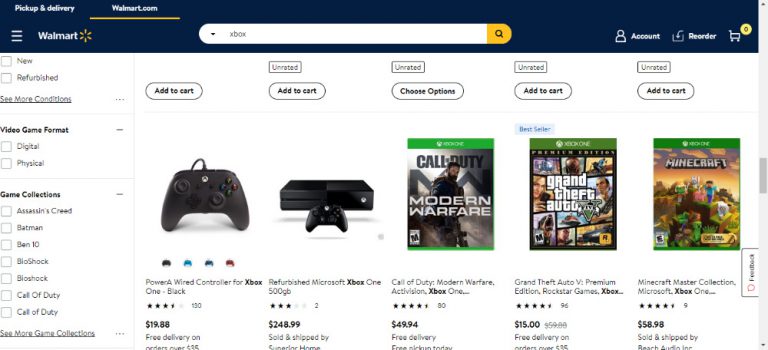In this image of a Walmart online shopping page, the top section is characterized by a blue banner. On the top left, there is white text reading "Pickup & Delivery," and beside it, "Walmart.com" with a yellow underline. Below this banner, on the left, are three horizontal lines followed by the Walmart logo. Centrally located is a search bar pre-filled with the word "Xbox," featuring a yellow magnifying glass icon to its right. Adjacent to this are icons for account access, reorder options, and a shopping cart with a zero inside a circle next to it.

Beneath the header, a left sidebar presents filter options. The "Condition" filter includes checkboxes for "New" and "Refurbished," with an option to see more conditions indicated by an ellipsis. The "Video Game Format" filter offers checkboxes for "Digital" and "Physical." A "Game Collections" section lists titles such as Assassin's Creed, Batman, Ben 10, BioShock, and Call of Duty, with an option to see more collections.

The main body of the page appears with a white background. It features several prominent listings, each with actionable white buttons. The top listings display "Add to Cart" or "Choose Options" accompanied by an unrated box.

Highlighted products include:

1. **PowerA Wired Controller for Xbox One (Black)**:
    - Image of a black Xbox controller.
    - Rating: 4.5 stars (30 reviews).
    - Price: $19.88.
    - Note about free delivery on orders over $85 (partly cut off).

2. **Refurbished Microsoft Xbox One 500 GB**:
    - Rating: 3 stars (2 reviews).
    - Price: $248.99.
    - Sold and shipped by Superior Home (partly cut off).

3. **Call of Duty: Modern Warfare (Xbox One)**:
    - Cover art visible.
    - Rating: 4.5 stars (8 reviews).
    - Price: $49.94.
    - Options for free delivery and free pickup available.

4. **Grand Theft Auto V: Premium Edition (Xbox)**:
    - Cover art visible.
    - Rating: 4.5 stars.
    - Price: $15.00 (discounted from $59.00).
    - Free delivery on orders over $85.

5. **Minecraft Master Collection (Xbox One)**:
    - Cover art visible.
    - Rating: 4.5 stars (9 reviews).
    - Price: $58.98.
    - Sold and shipped by Beach Audio.

This detailed depiction captures the structure, key elements, and specific product listings, giving a comprehensive overview of the Walmart shopping page for Xbox-related items.